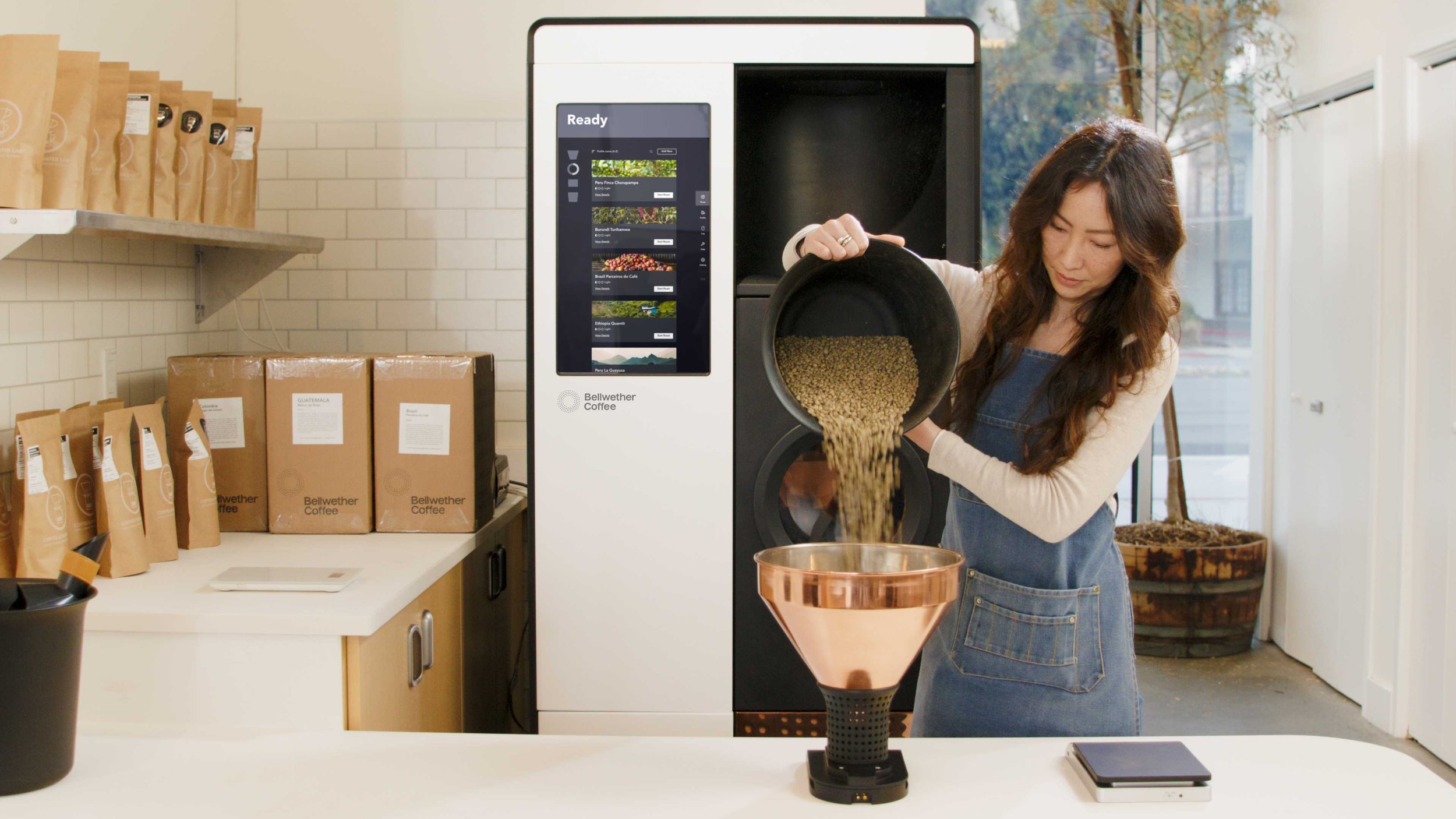The color photograph is captured in a landscape orientation, portraying a detailed and realistic scene of a woman in her 30s standing on the right side. She is engaging with a measuring device on a countertop directly in front of her. Carefully, she pours light-colored beans, possibly coffee beans, from a gray bucket into a copper-hued, pyramid-shaped measuring container. This container is wide at the top and narrows towards a black base. The woman is dressed in a blue denim apron paired with a long-sleeved white top, and her long, curly dark hair cascades down her back.

In front of her on the counter, to the right, lies a black notebook. Dominating the background is a stainless steel vending machine with a black section on its right side and various selection buttons at the top left. The left side of the photograph features a storage counter cluttered with several brown shipping boxes and bags, all adorned with white labels, though their texts are unreadable. The overall style of the photograph falls under photographic representationalism realism, emphasizing a lifelike depiction of the scene.